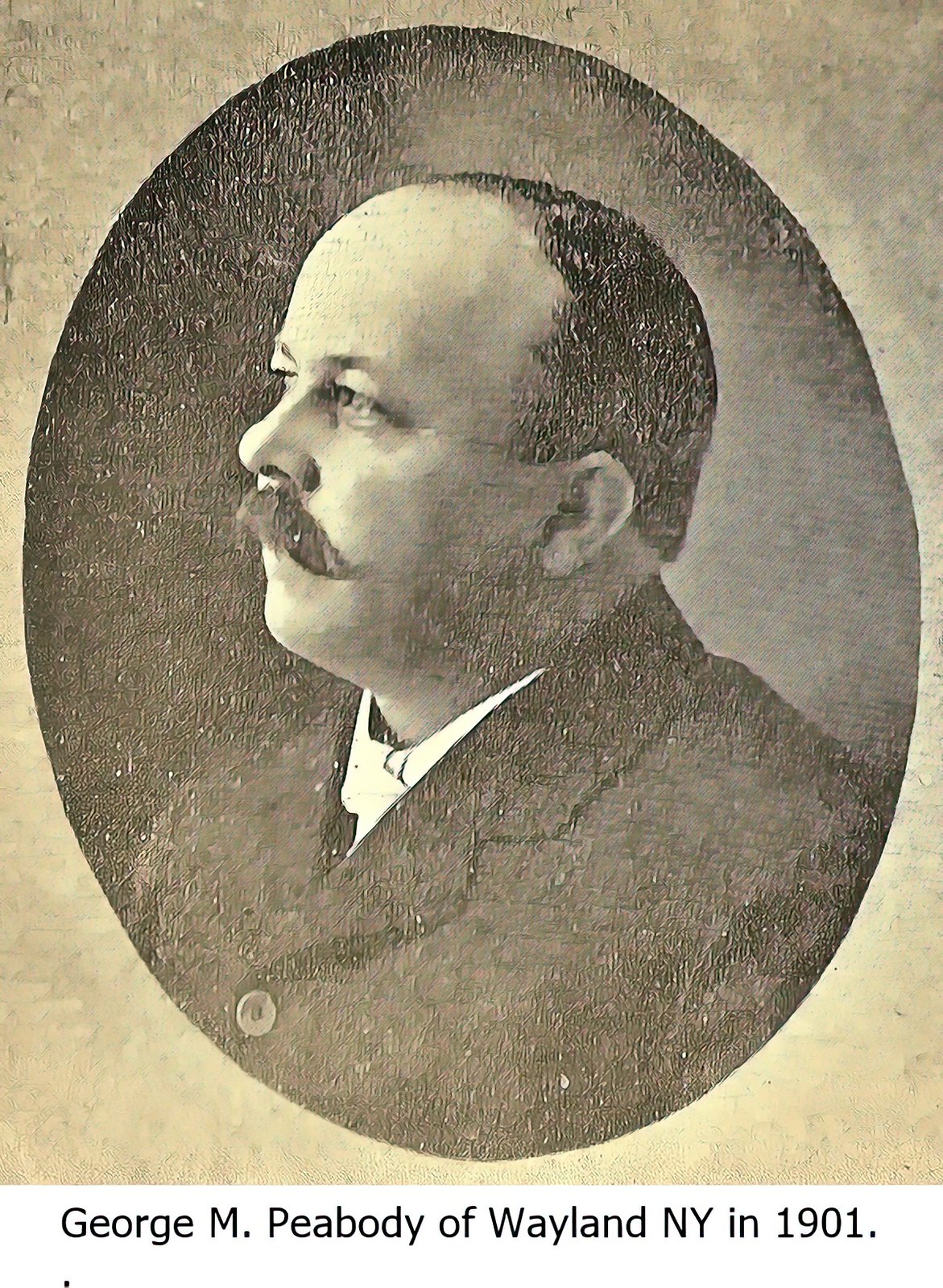This black and white portrait features George M. Peabody of Wayland, New York, in 1901. The photograph is centered within a dark gray or black oval, set against a light gray or beige background. George is dressed in a buttoned-up black or dark suit jacket, with a hint of a white collared shirt visible at the neckline. His short hair, which appears black or brown, is receding at the front. He sports a handlebar mustache and is posed in profile, facing the left side. Beneath the portrait, black text reads, "George M. Peabody of Wayland, NY in 1901."